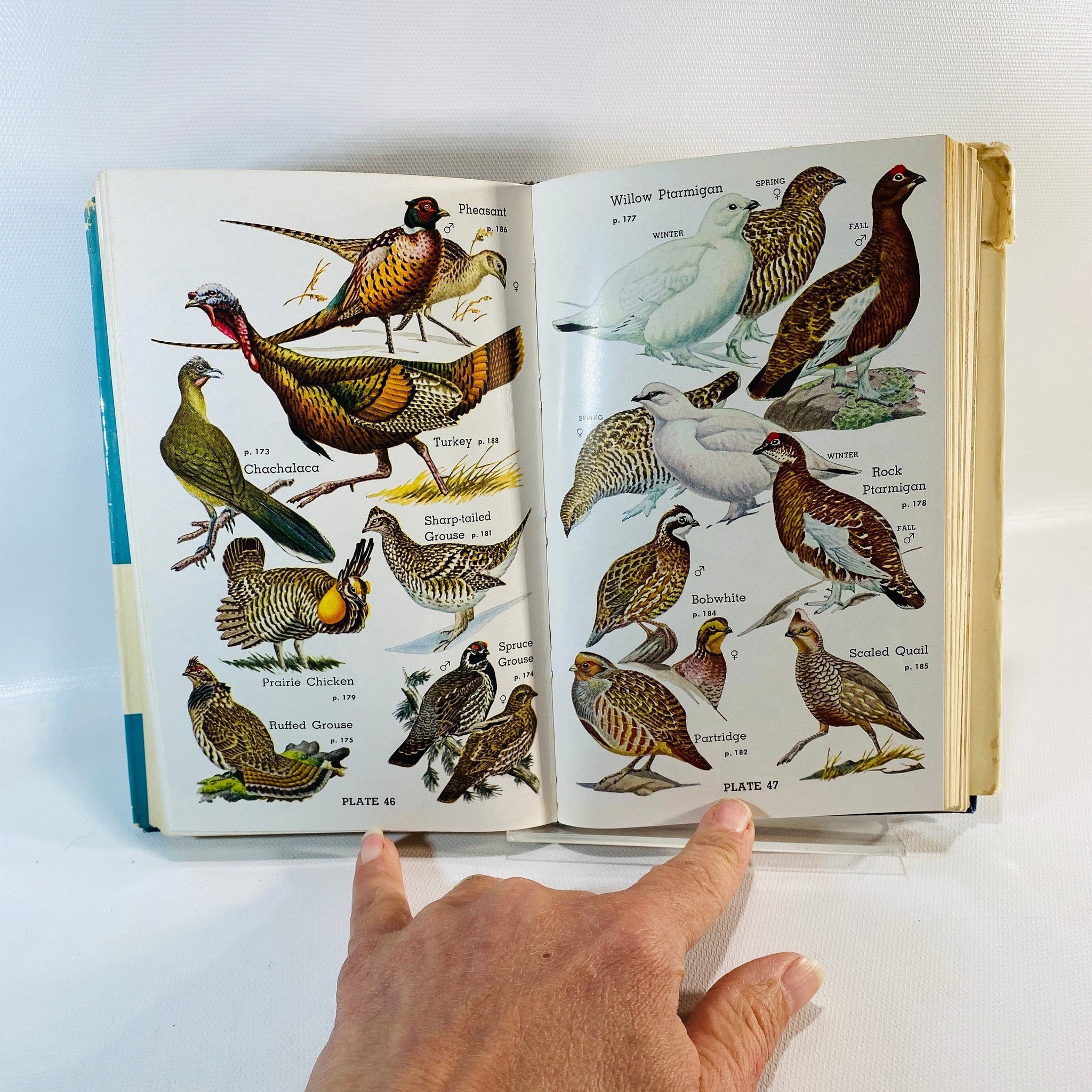In this captivating image, we see a vintage-style book opened and displayed against a pristine white backdrop. A Caucasian individual’s hand is prominently featured at the bottom of the image, with the pinky and index fingers extended to keep both pages of the book open. The pages are richly adorned with detailed illustrations of various bird species.

On the left-hand page, labeled "Plate 46" at the bottom, the colorful depictions include a pheasant, a turkey, a chachalaca, a sharp-tailed grouse, a prairie chicken, a spruce grouse, and a ruffed grouse. These illustrations burst with life through the use of hues that range from vibrant reds and oranges to more muted browns and greens.

The right-hand page, marked "Plate 47" at the bottom, showcases an equally diverse set of birds including a white ptarmigan, a rock ptarmigan, a bobwhite, a scaled quail, and a partridge. Each bird is meticulously drawn, capturing the essence of their unique plumage with shades of white, brown, yellow, and green interspersed with splashes of red and orange.

Overall, this image artfully combines the elegance of hand-drawn ornithological illustrations with the timeless appeal of a vintage book, creating a visually arresting and informative tableau.